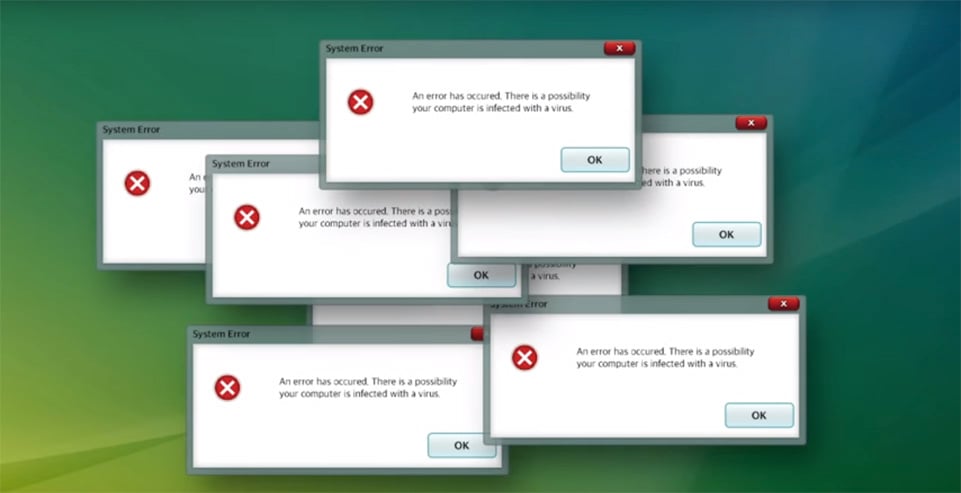This image captures a chaotic computer desktop with seven overlapping error pop-up messages dominating the center of the screen. Each rectangular pop-up, prominently displayed in the middle, features a red X icon on the left and a message stating, "An error has occurred. There is a possibility your computer is infected with a virus." Each pop-up also includes an OK button for acknowledgment and a red X in the top right corner for closing the window. The errors are arranged in an overlapping pattern, spreading from the top center and cascading towards the lower right and left, creating a cluttered and chaotic appearance. The backdrop of the screen features a distinctive gradient, starting from a bright yellowish-green in the bottom left corner, transitioning to a deep hunter green in the bottom right, and blending into a bluish-green in the top right. This gradient provides a stark contrast to the white backgrounds of the error messages, emphasizing the disordered nature of the screen and the possibility of a virus infection.